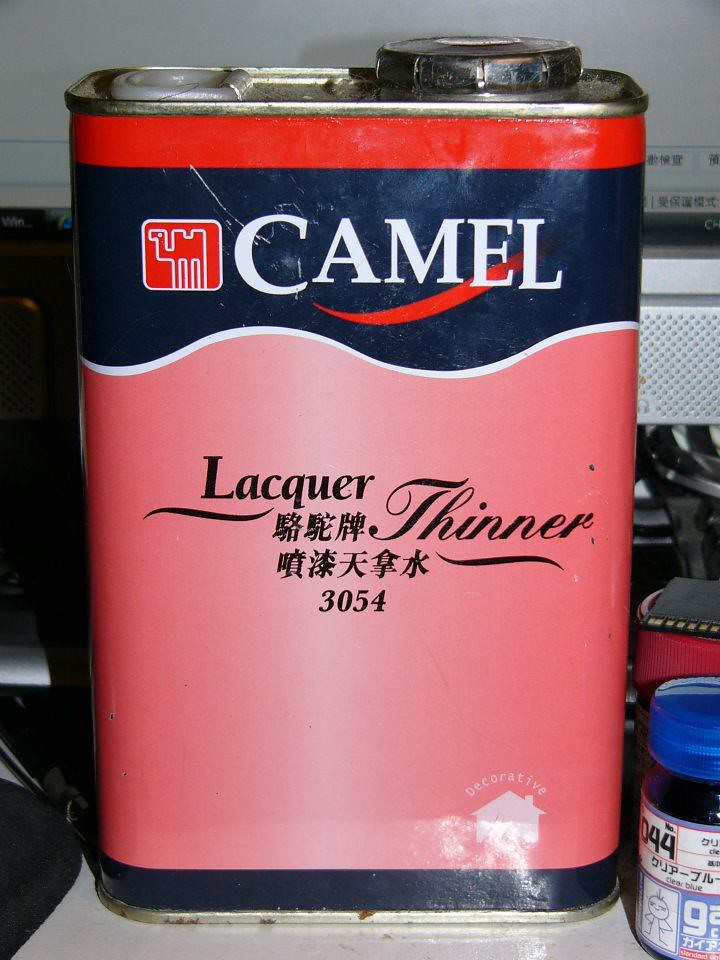This vertically-oriented photograph showcases a tin can positioned on a flat surface such as a counter, shelf, or table. The can, which is rectangular in shape, features a distinctive red, blue, and white label. At the top of the can, a twistable spout is visible, reminiscent of those used to pour transmission fluid or oil. The label prominently displays the word "camel" in white text, accompanied by an illustration of a camel in red and white. Below this, against a light red background, the blue text reads "Lacquer Thinner 3054." The label also includes several lines of Asian script, indicating cultural origins that are not further identifiable by the observer.